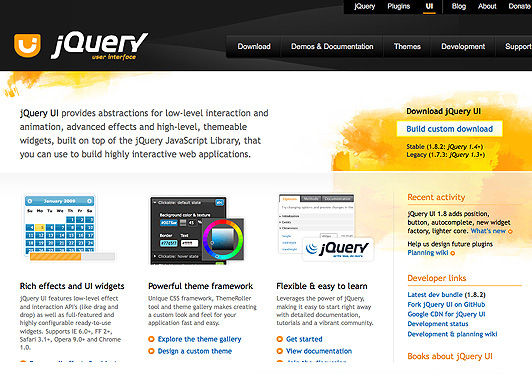This is a cropped screenshot of a website's homepage, featuring a distinct black header adorned with a unique design. At the bottom of the header, there's a rounded, light grey object, and to the right, a darker grey object that combines rounded and sharp corners.

On the left side of the header is an orange, rounded shield-shaped icon with a white 'U' in the center, where the top right of the 'U' is a white square. Adjacent to this icon is the "jQuery" logo, where the left fork of the 'Y' is partially obscured by the top of the 'R.' Below this logo, in smaller, orange italicized text, is the phrase "user interface."

To the right of the "jQuery" logo are several buttons with a gradient background transitioning from black to light grey and featuring white text. The buttons are labeled, from left to right: "Download," "Demos and Documentation," "Themes," "Development," and "Support." Above this set of buttons is a smaller menu with different white text labels which include: "jQuery," "Plugins," and "UI," with "UI" underlined in orange. A vertical white line separates this mini-menu from additional links: "Blog," "About," and "Donate."

Beneath the header, the webpage's body features a primarily white background accented with orange and yellow splotches in the top left and along the right-hand side. In the top left of the body section, there is a paragraph of black text.